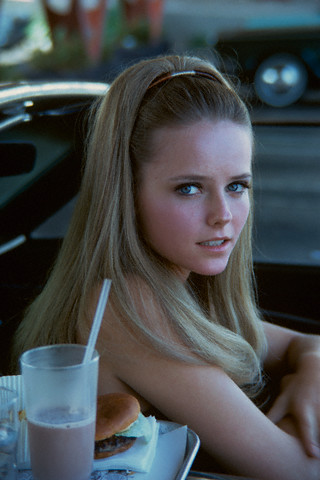In this vintage photograph, likely from the 1960s or 70s, a young woman with striking blue eyes and long blonde hair is seated in a black convertible. Her hair is pulled back by a headband adorned with brown, white, and orange stripes, lending a distinct retro flair to her look. She exudes a timeless beauty, evoking the style of a model or actress from that era.

The setting appears to be a classic drive-in restaurant. Perched on a metal tray next to her is a half-drunk chocolate milkshake with a straw and a cheeseburger topped with a piece of lettuce. The ambiance captures an iconic American feel, reminiscent of scenes from movies like American Graffiti. In the distance, a blurred-out car adds to the nostalgic atmosphere, while her serious, somewhat annoyed expression adds a layer of depth to the image, suggesting a story behind her poised exterior.